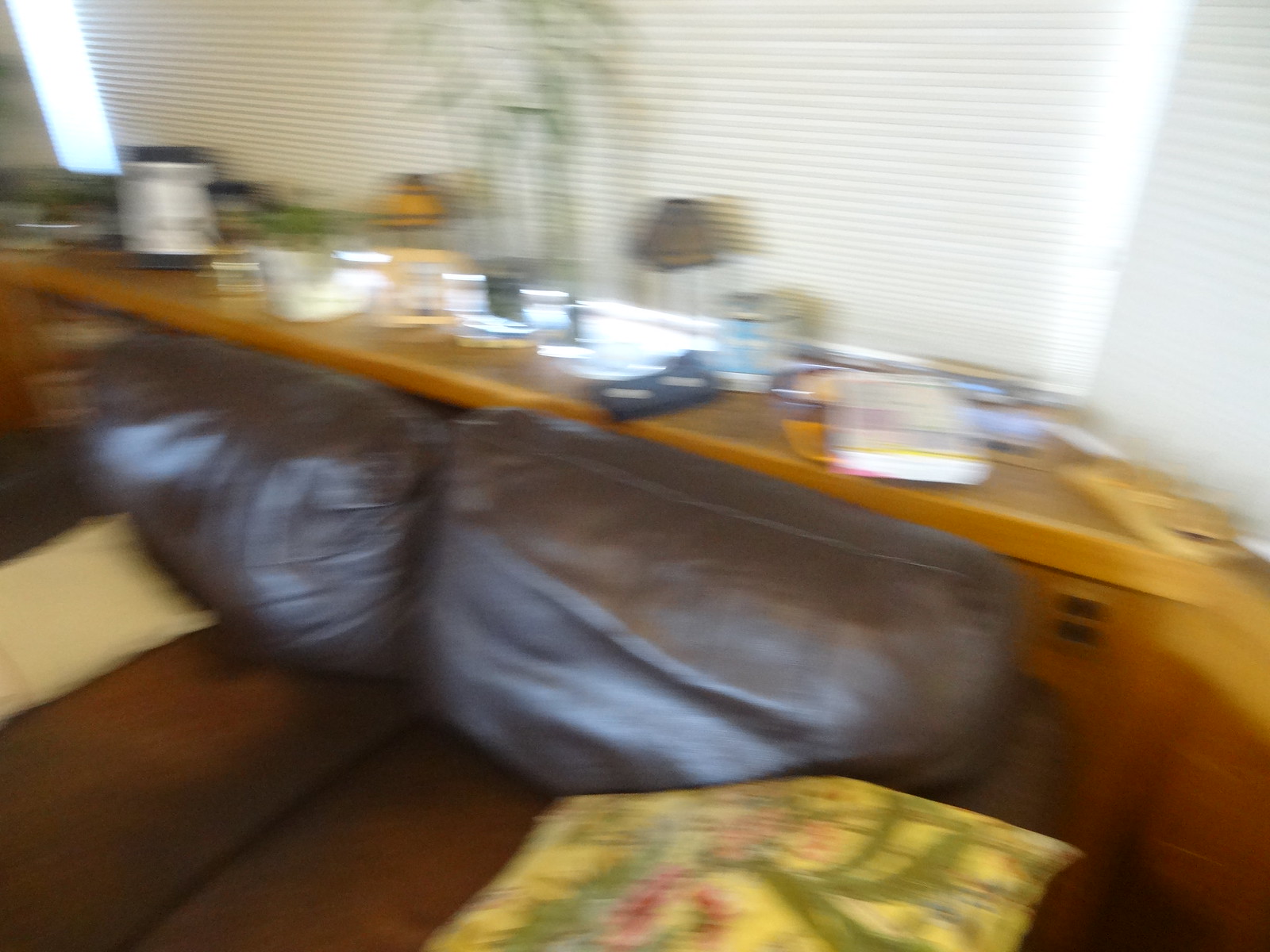This photograph, albeit slightly blurry, captures a cozy corner within a house. The image prominently features a series of windows stretching horizontally from the left to the right across the upper part of the frame. These windows are adorned with white lines, presumably frames or blinds, which are currently closed.

Directly beneath the windows, there's a narrow countertop adorned with an array of eclectic items. Taking center stage is a verdant plant that adds a touch of nature to the scene. Flanking the plant are several diminutive lamps with petite lampshades, lending a warm and inviting ambiance. Scattered alongside are a few books, and intriguingly, there appears to be an old VHS tape among the assortment, hinting at a nostalgia-tinged personal space.

Below the countertop, several brown bean bags are casually arranged, suggesting a comfortable and informal seating area. Towards the right side of this lower section, there is a yellow item, adorned with a floral pattern. It's unclear whether this item is a bag or a pillow, but its bright color and decorative design certainly catch the eye, contributing an additional layer of homeliness and charm to this inviting interior scene.